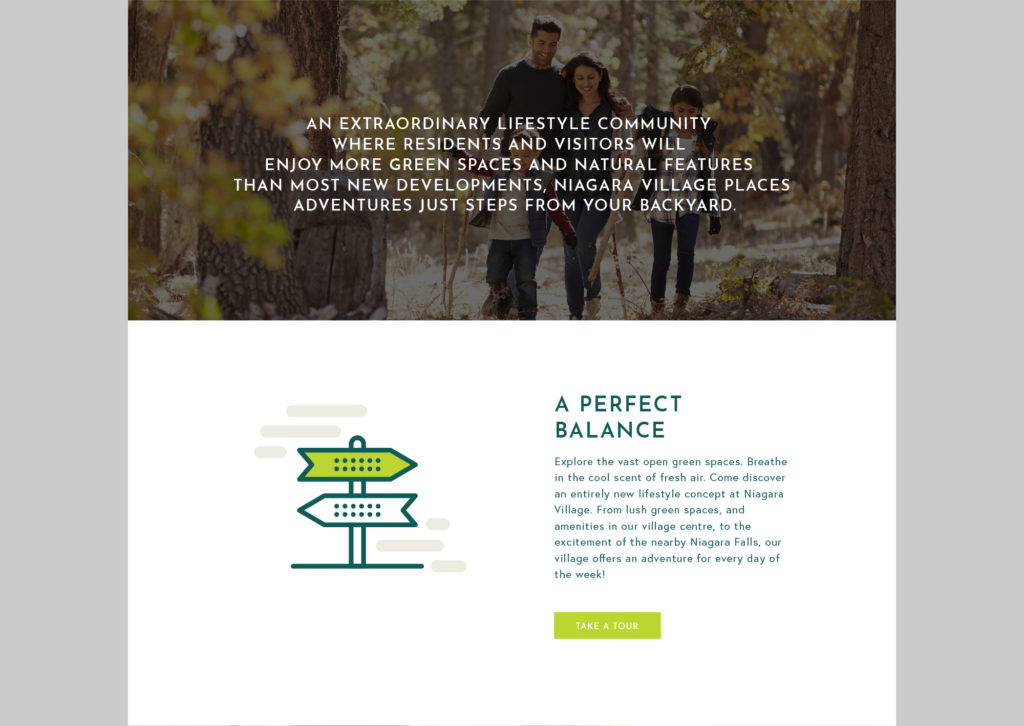In this charming, woodland scene, a couple is seen playing with their children amidst the backdrop of a serene forest. Majestic trees with lush, green leaves surround them, creating a natural canopy. The accompanying text extols the virtues of Niagara Village, an extraordinary lifestyle community that promises residents and visitors a greener, more nature-connected existence compared to most new developments. Here, adventures are just steps from your backyard. This idyllic setting offers a perfect balance between vast, open green spaces and modern amenities. Visitors are encouraged to breathe in the fresh, cool air and discover a unique lifestyle concept at Niagara Village. From the lush greenery and village center amenities to the thrill of nearby Niagara Falls, this community provides an adventure for every day of the week.